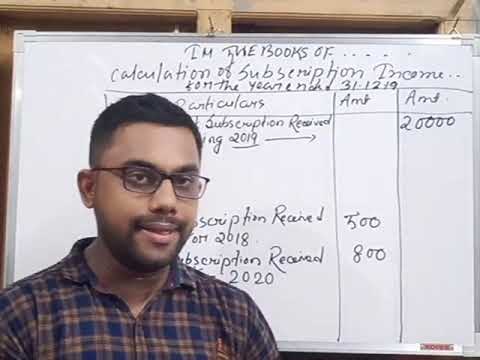In the image, a young man with light brown skin stands in front of a whiteboard. He has short cropped black hair and is sporting a mustache and beard. He wears prescription glasses and a blue and brown plaid button-up shirt. His lips are slightly parted, capturing him mid-sentence, likely as he explains information written on the whiteboard behind him. The text on the whiteboard, which appears handwritten using markers, includes phrases like "in the books of calculation of subscription income," alongside listed monetary amounts such as $500, $800, and $20,000. Additional text includes "subscription received 2018" and "subscription received 2020." The setting and context suggest that he is delivering financial advice, perhaps during a lecture or a video call, with the focus on explaining a table of subscription income data.